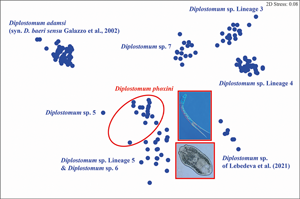This image appears to be an extremely small and illegible diagram or cropped section from a research article, textbook, or PowerPoint presentation slide. It features a black line around a white background, with text in dark blue that remains unreadable despite magnification due to severe distortion. Scattered throughout the image are dark blue blotches, as if ink has spilled. Notably, there are two images outlined in red: one in portrait orientation displaying a blue swatch with a diagonal white line, and another in a square format showing an indistinct gray object against a lighter background. Additionally, some areas with dark blue ink dots are circled in red, hinting at a focus or a point of interest. The top portion of the image faintly suggests the text "2D source," adding to the academic or technical nature of the content.